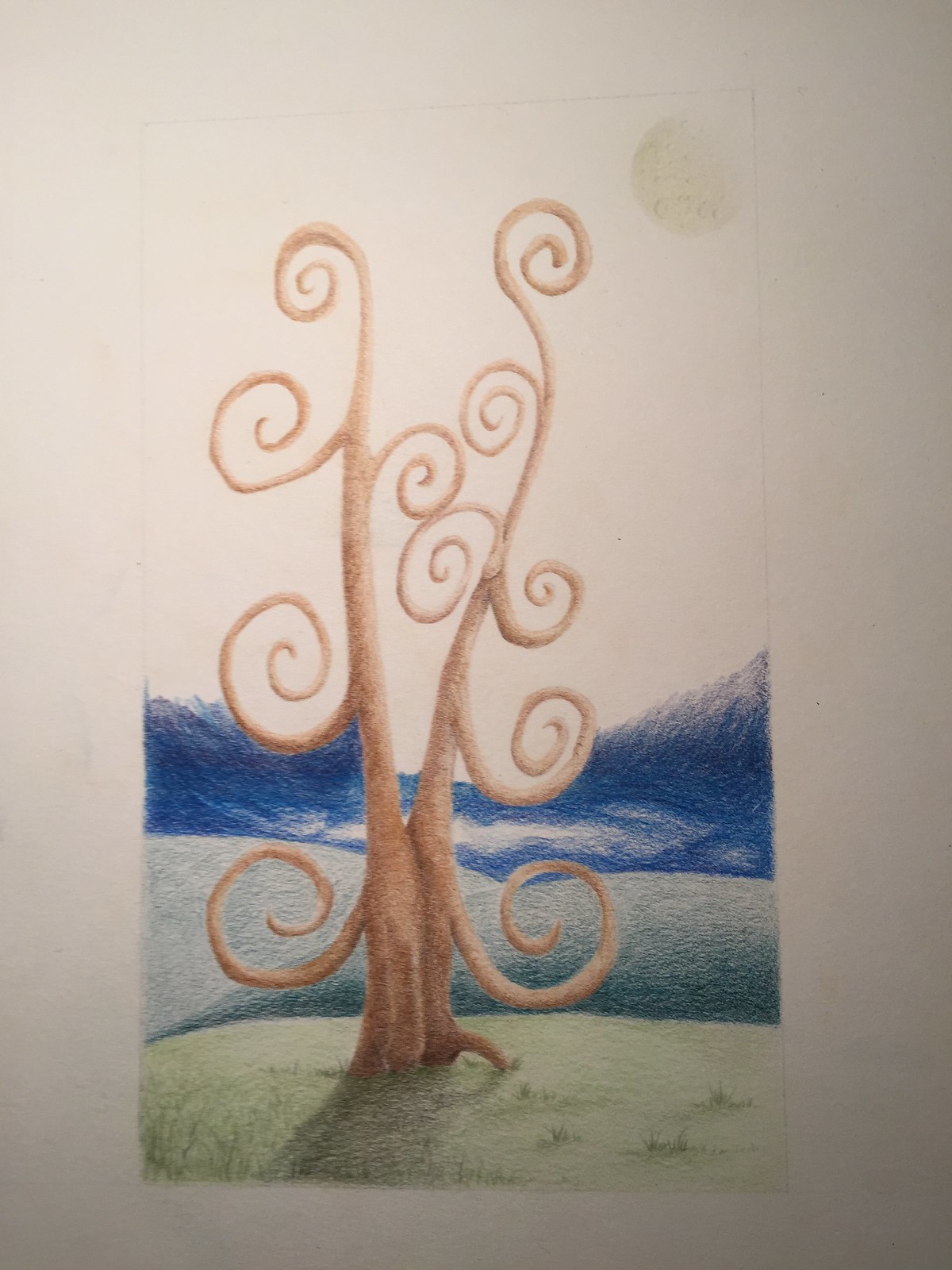Here is a detailed and cleaned-up caption for the image described:

---

A whimsical artwork captures a fantastical scene, framed in a gray background and viewed slightly from the side, suggesting an image of some sort of painted canvas or paper. Central to the picture is a serene, white backdrop that sets the stage for a vibrant, yellow moon nestled in the top right corner. Midway down the canvas, a serene blue ocean melds with rolling blue hills, eventually transitioning into a blue grassy expanse. Dominating the foreground is a playful, peachy-pink tree that stretches almost to the moon. The tree elegantly splits into two main branches. The left branch features four distinct, curved offshoots while the right side displays three. Each offshoot delicately mimics squiggles, creating an impression of whimsical branches that enhance the fanciful nature of the piece.